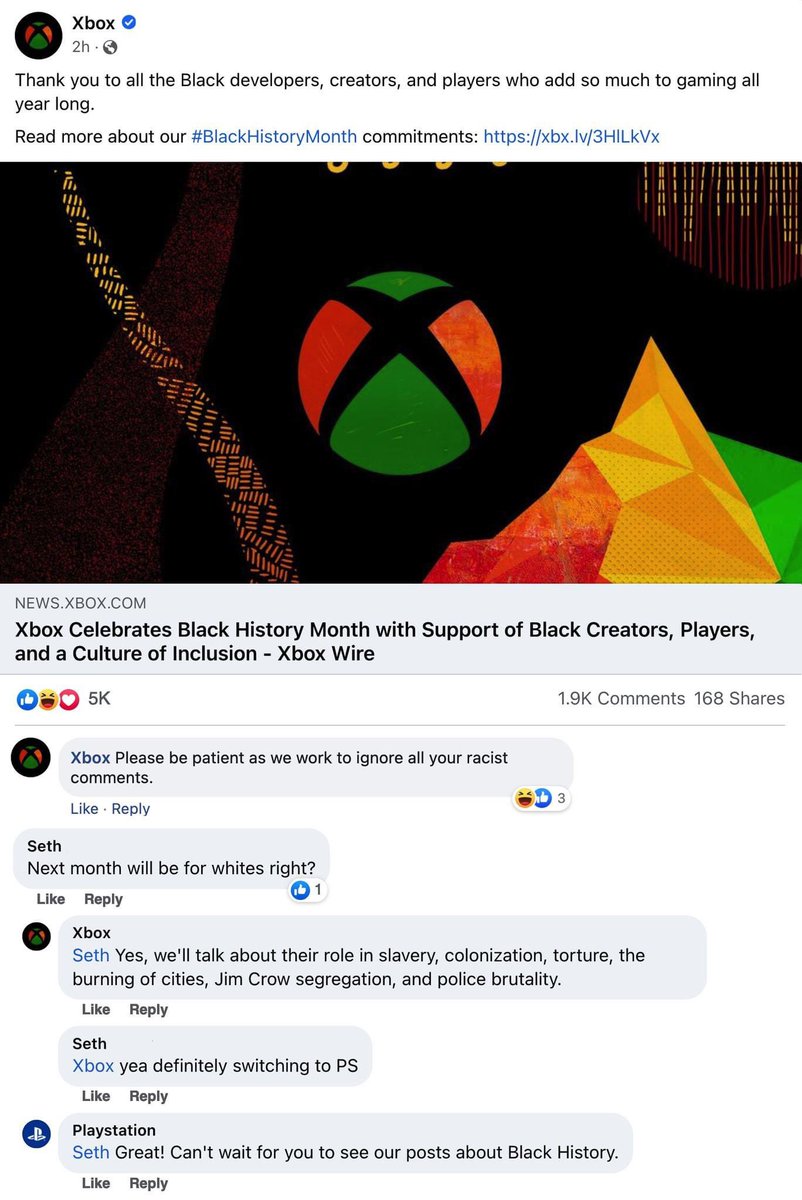The image captures a social media post from Xbox, set against a white background. At the top, there is a circular graphic representing the user's profile picture, adjacent to which is the Xbox logo. A blue circle with a white check mark is also present, indicating verification. 

Below these elements, in black text, the message reads: "Thank you to all the Black developers, creators, and players who add so much to gaming all year long. Read more about our Black history." This message is followed by the hashtag "#BlackHistoryMonth" in blue text. 

There is also a blue link directing to Xbox's website. The subsequent graphic features a black background accented with digital stripes, and a prominent green 'X' surrounded by an orange border. The heading "Xbox celebrates Black History Month with support of Black creators, players, and a culture of inclusion," followed by "Xbox Wire" appears below the image.

Engagement icons including a like symbol, a laugh symbol, and a heart symbol show the post's popularity with "5K likes," "1.9K comments," and "168 shares." The comments section transitions back and forth between responses from Xbox and various users.